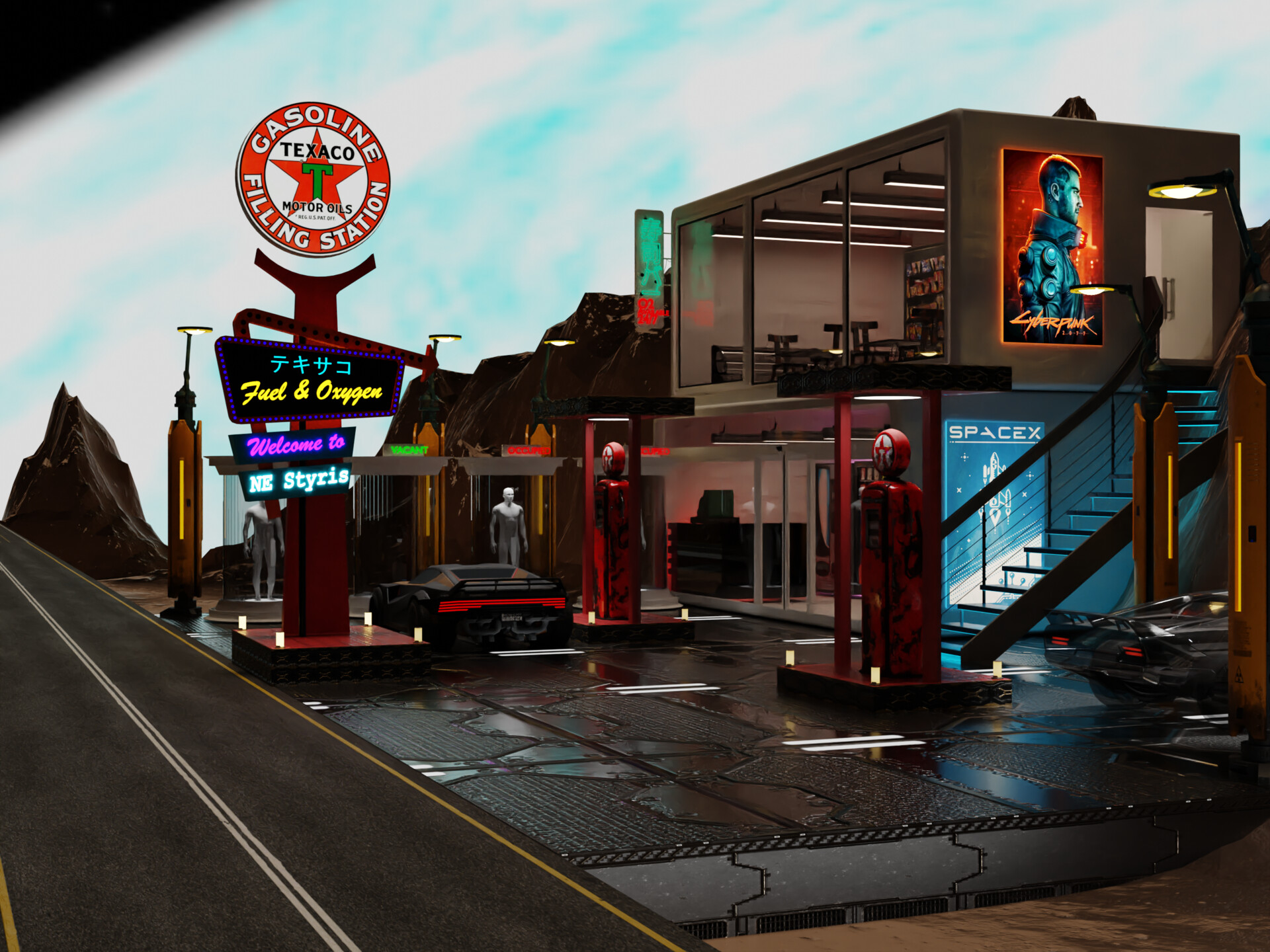This image captures a striking scene of a modern, cyberpunk-themed Texaco fueling station situated beside a road. The focal point is a two-story rectangular building located on the right-hand side. The building boasts large glass panels across both floors, giving it a sleek, contemporary appearance. Metal stairs lead to the second floor, which features bar stools and high-top tables, adding a unique social element to the location.

In front of the building, there are classic red Texaco gas pumps, easily recognizable by their vintage glass globes and red stars. Adjacent to the pumps are futuristic, black Lamborghini-style cars with distinctive long red lights. A glass staircase on the side adds to the building's modern aesthetic.

Prominent signage includes a blue glowing sign with a spaceship, labeled "Space X," adding to the cyberpunk vibe. Another large red sign features Japanese text, "Fuel and Oxygen," and welcomes visitors to Nestyrus. At the top of this sign is a red circular emblem that reads "Gasoline Texaco Filling Station," emphasizing the retro-futuristic blend of elements. Adding to the ambiance, there's a poster on the top floor depicting a man and the word "Cyberpunk." The fusion of modern architecture, vintage Texaco branding, and futuristic elements creates a visually compelling and richly detailed scene.